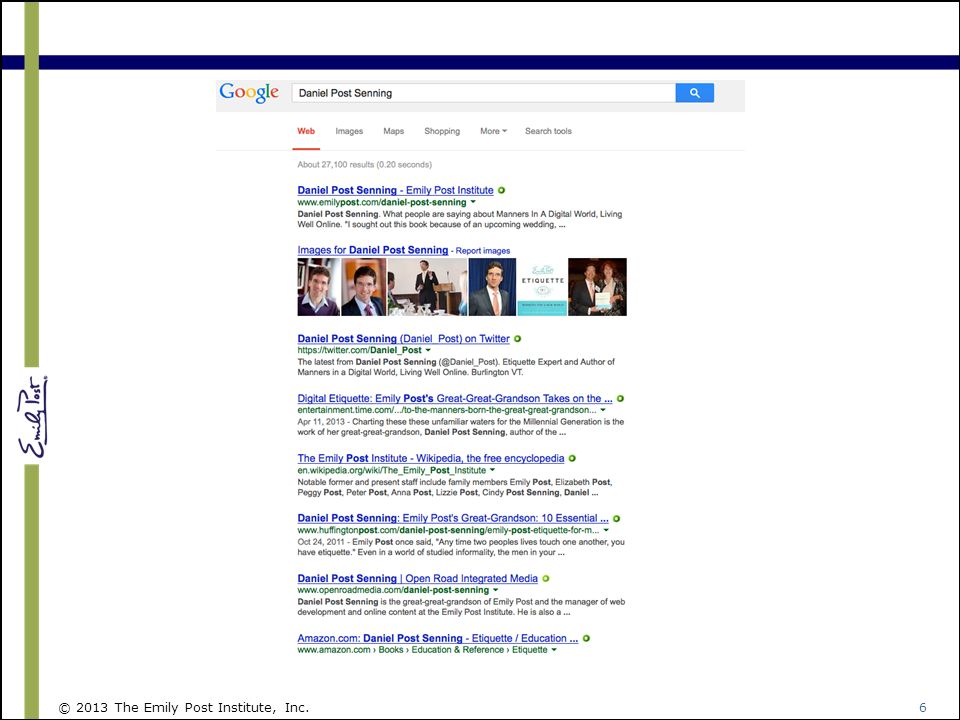The image depicts a detailed Google search results page for "Daniel Post Sending." At the top, a deep blue horizontal bar spans from left to right, and a green vertical bar extends from the bottom to the top, originating in the left-hand corner. The green bar features some handwritten text, potentially indicating "Emily Post," although it is somewhat illegible.

Below the blue bar, the familiar Google search bar is visible, displaying the search query "Daniel Post Sending" and a search button. Beneath this, a row of selectable options reads: Web, Images, Maps, Shopping, More, and Search Tools. The search results indicate about 27,100 results were found in 0.20 seconds.

The first search result is a link to the Emily Post Institute, with a snippet mentioning "Daniel Post Sending" and the book "Manners in a Digital World: Living Well Online." The link elaborates on a personal search for the book, possibly in relation to an upcoming wedding. Following this, there is a section labeled "Images of Daniel Post Sending," featuring about five or six profile pictures of a man in a suit.

The subsequent result is "Daniel Post Sending, Daniel_Post on Twitter," followed by a brief description. Additional clickable links include "Digital Etiquette: Emily Post's Great-Grandson Takes On...," "Emily Post Institute - Wikipedia, the free encyclopedia," and "Daniel Post Sending: Emily Post's Great-Grandson, 10 Essential..." with smaller descriptive text under each. Further down, "Daniel Post Sending, Open Road Integrated Media," and "Amazon.com: Daniel Post Sending: Etiquette / Education" are noted.

At the very bottom of the image, a footer reads "Copyright 2013, Emily Post Institute, Inc."